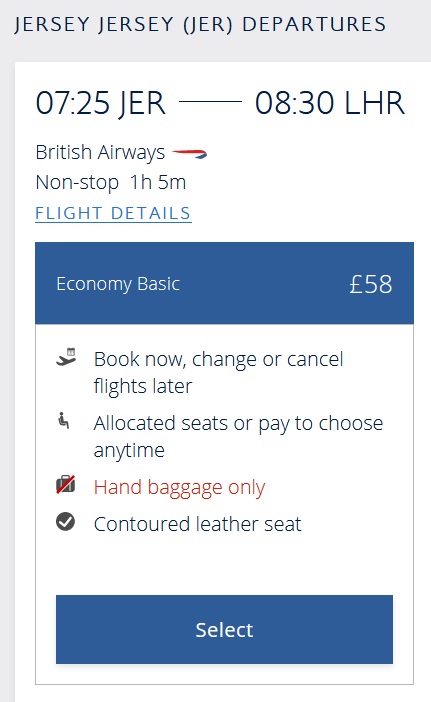Screenshot of flight information for a British Airways journey from Jersey to London Heathrow. The background is primarily white, with a light gray bar at the top and along the left side. In the gray bar, it reads "Jersey, Jersey (JER) Departures." The flight details include "072:25 JER – 08:30 LHR," indicating the flight time. The journey is non-stop, lasting one hour and five minutes. Below, in blue and underlined, there's a clickable link labeled "Flight Details."

Highlighted within a blue background, "Economy Basic, £58" is stated. Further details on a white background include options to "Book Now, Change or Cancel Flights Later," and mention that seats can be allocated or chosen for a fee anytime. In red text is the note "Hand Baggage Only," with subsequent information about a "Contoured Leather Seat" included. A blue bar at the bottom displays a white "Select" button.

This screenshot likely serves as a reference for someone looking up or booking flight information.